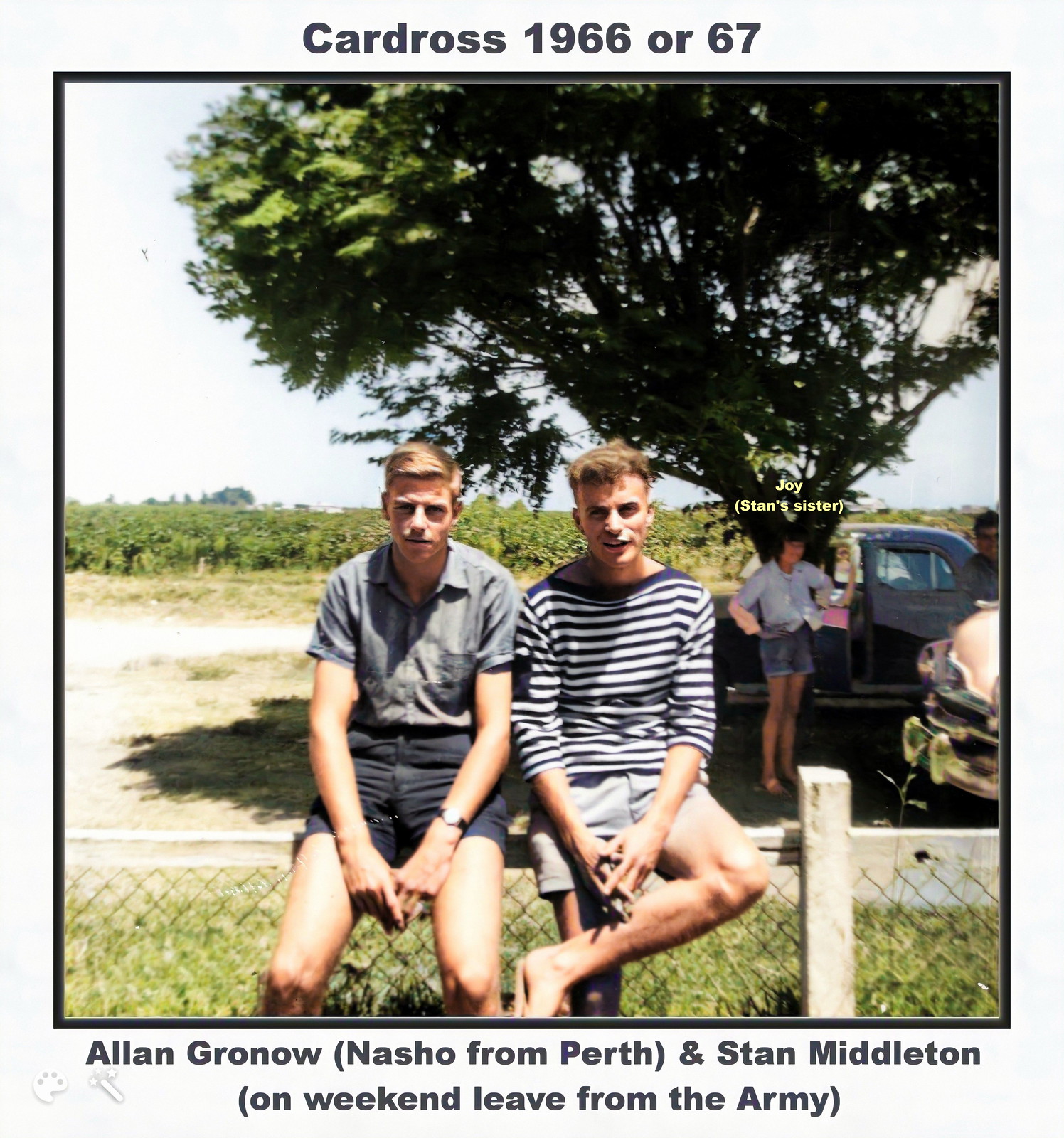This is a color photograph taken outdoors in Cardross around 1966 or 1967. The top caption reads "Cardross 1966 or 67" and below it, the accompanying text identifies the individuals as Alan Grosh from Perth and Stan Middleton on weekend leave from the Army. The scene includes two young men, appearing to be about 18 years old, sitting on the top railing of a small fence. Both have short brown hair, parted on the side, and are dressed in short-sleeve shirts and shorts, fitting with the warm day suggested by the partly blue sky and scattered white clouds.

One of the young men sports a plain button-down shirt and has a pensive expression, while the other, wearing a striped pullover shirt, has a half-smile. Their postures differ, with one individual sitting with legs spread and hands parked on his legs, while the other has one leg crossed over the other. A lush green lawn is visible through the fence they sit on, and a large tree stands in the background, adding to the serene, summery atmosphere.

Additionally, in the background to the right, a young lady identified as Joy, Stan’s sister, is seen standing near a vintage 1950s truck.